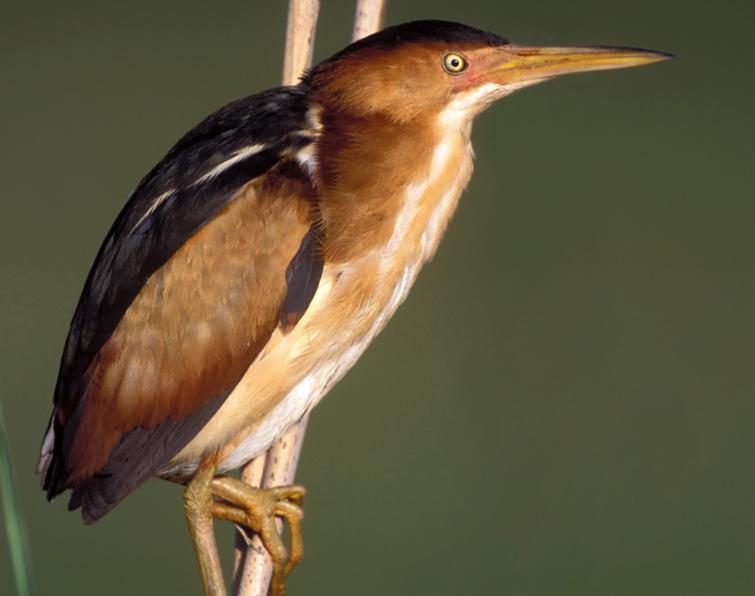This is a close-up, landscape-oriented photo of a colorful bird perched slightly left-of-center on thin, vertical branches, with one foot placed above the other. The bird faces right, displaying its remarkable plumage. Its head is adorned with a dark reddish brown on top that extends into black further back, while its face and cheeks feature a shiny light brown. It boasts a prominent, long, yellow beak with a black tip, complemented by a bright yellow eye. The bird's chest and underside are streaked with white and very light brown, contrasting with the dark, almost black, back that shows some white streaks. The wings are black on top and light brown underneath, with the dark feathers meeting at the back. This bird grips the branches with visible yellow talons, with one leg stretching down out of the frame. The background is a subtle greenish-gray, providing a neutral backdrop that highlights the bird's vivid colors and intricate details.